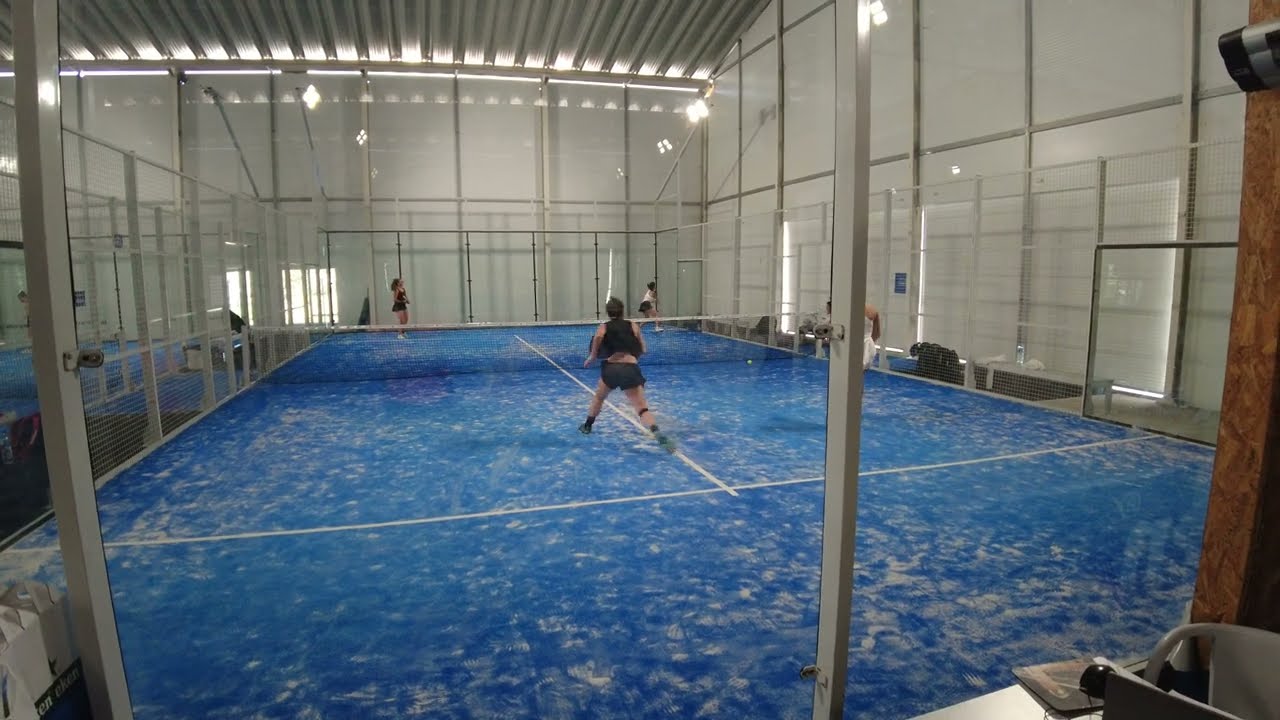This color photograph, captured in landscape orientation, reveals an indoor racquet sport court enclosed by glass walls. The court, featuring a blue surface marked with a white perpendicular and parallel grid, suggests a sport like squash or racquetball rather than tennis. From a vantage point in a viewing area, we observe three players on the court: one in the near court and two in the far court. The central player is distinctly wearing a black outfit with leg straps. Reflections and window frames partially obscure the scene, yet the net in the middle is clearly visible. The photograph also captures peripheral details such as a ladder leaning against a wall to the right, a high ceiling with several lights, and a commercial-style steel corrugated roof, enhancing the atmosphere of a gym or workout facility. The realistic, representational style of the photograph underscores the dynamic setting and activity within the enclosed court.